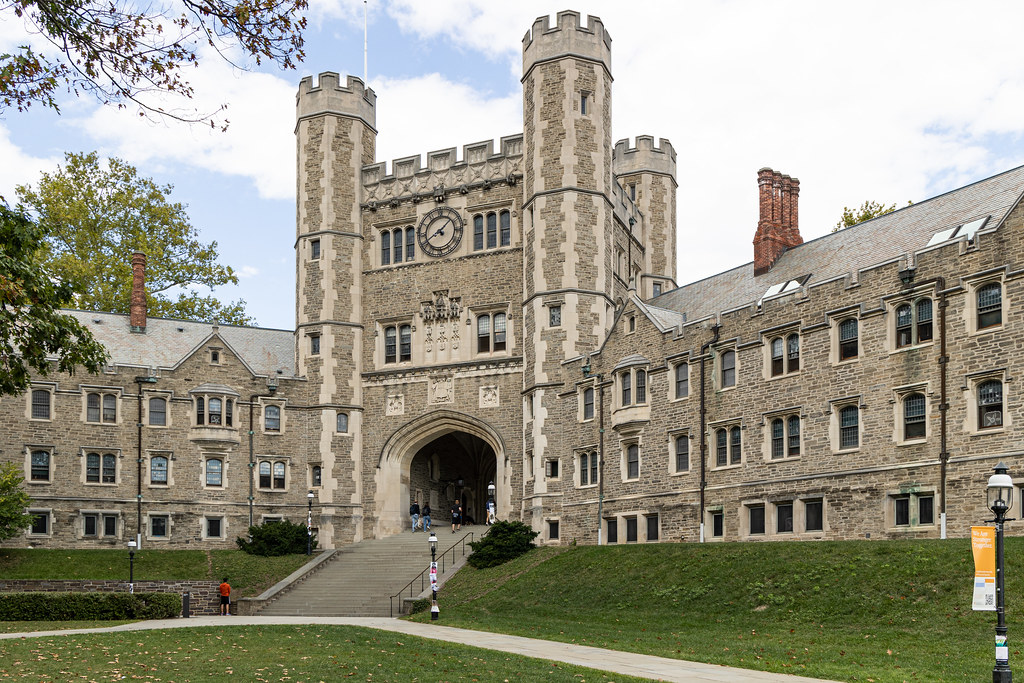This color photograph captures the entrance to an impressive academic building, likely on a college campus. The structure, crafted from brown stone with light stone trim, has a striking, castle-like aesthetic. It features a central tower topped with crenellations and a prominent black metal clock set against a stone background. The building is flanked by two identical extensions, both adorned with gray roofs, numerous windows, and brick chimneys with multiple outlets.

At the base of the central tower lies a large archway, which opens to a stairway descending to a grassy slope. The sidewalk at the bottom of the slope meanders through a well-manicured lawn, dotted with a few shrubs, leading up to the stairs. Pedestrians can be seen walking along the pathway and ascending the stairs, suggesting an active campus environment.

The scene is framed by a vibrant blue sky with scattered white clouds, and there are trees visible in the upper left-hand corner of the image, enhancing the picturesque quality of the setting. To the right of the staircase, near the tower, stands a signage pole, adding to the campus-like atmosphere. Overall, the photograph exudes a sense of historical elegance and liveliness on a beautiful day.